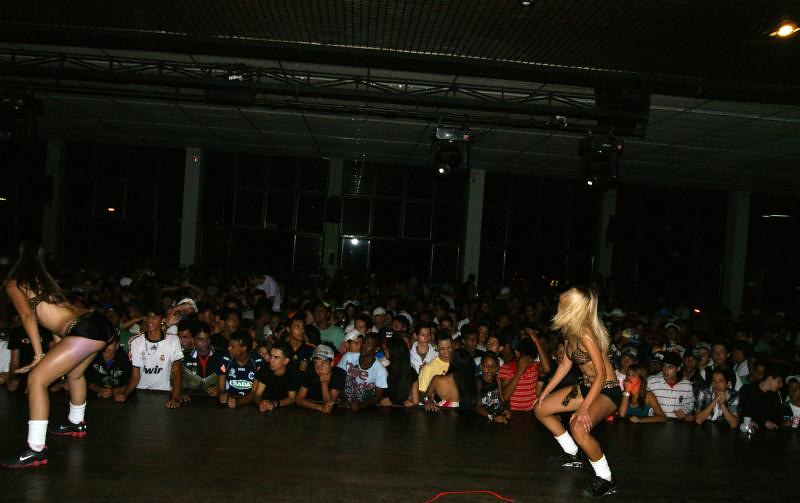The image depicts a lively, nighttime scene in a large building with numerous windows and structural beams. On a well-lit stage with a wooden floor, two scantily clad women are performing a provocative dance. The woman in the front is blonde, wearing a black bikini top, very short black shorts, white socks, and black shoes that appear to be Nike. She is bent over in a suggestive position, eliciting the attention of the audience. Behind her, a brunette woman, similarly dressed in a bra top and short shorts, also wears white socks and black shoes, possibly Adidas. The brunette has her butt raised, prompting many men in the front rows to watch intently; some even have their elbows on the platform. The crowd, dominated by men with a few scattered women, is densely packed, almost five or six rows deep. The venue, possibly a performance hall or gym, features prominent white beams, attached speakers, and overhead floodlights, adding to the dramatic atmosphere of the event.